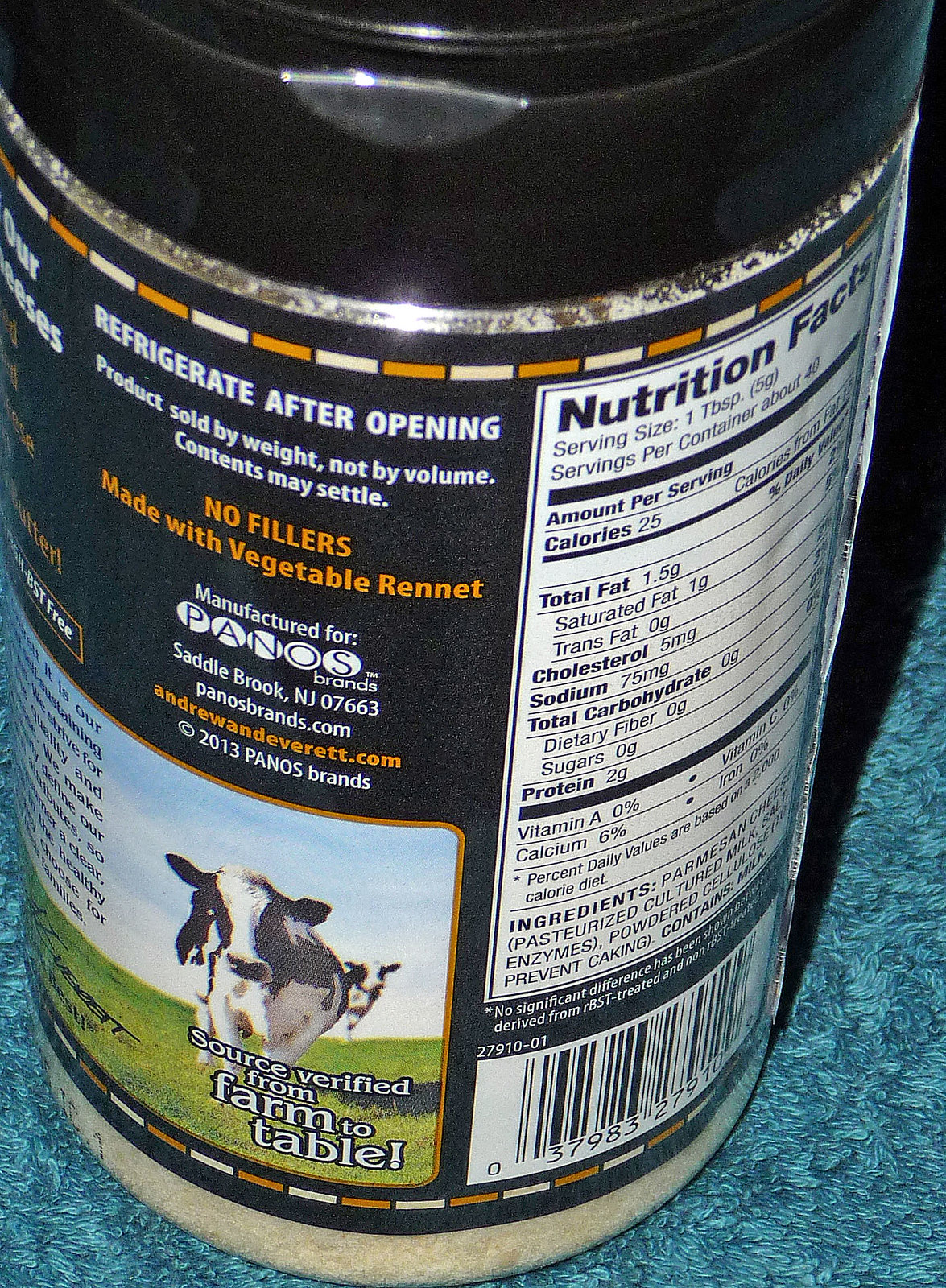The photograph showcases a food product with a distinctly designed black label featuring white and orange accents. The lower section of the label depicts an image of black and white cows grazing on lush green grass, accompanied by the phrase, "Source Verified from Farm to Table" in a bold white font. At the bottom part of the label, a black and white barcode with numerical identifiers is present. Additionally, a detailed nutrition facts section outlines the calories, fat content, and other ingredients in black and white text. 

The top portion of the label displays several important notices in white font, including, "Refrigerate After Opening," and "Product Sold by Weight Not by Volume, Contents May Settle." Just below these notices, in orange font, it states, "No Fillers, Made with Vegetable Rennet." The label also provides manufacturing details in white, indicating, "Manufactured by Panos Brands, Saddle Brook, New Jersey, 07663, panosbrands.com." Directly beneath this information, another web address is printed in orange, followed by a copyright date in white, noting the year 2013.